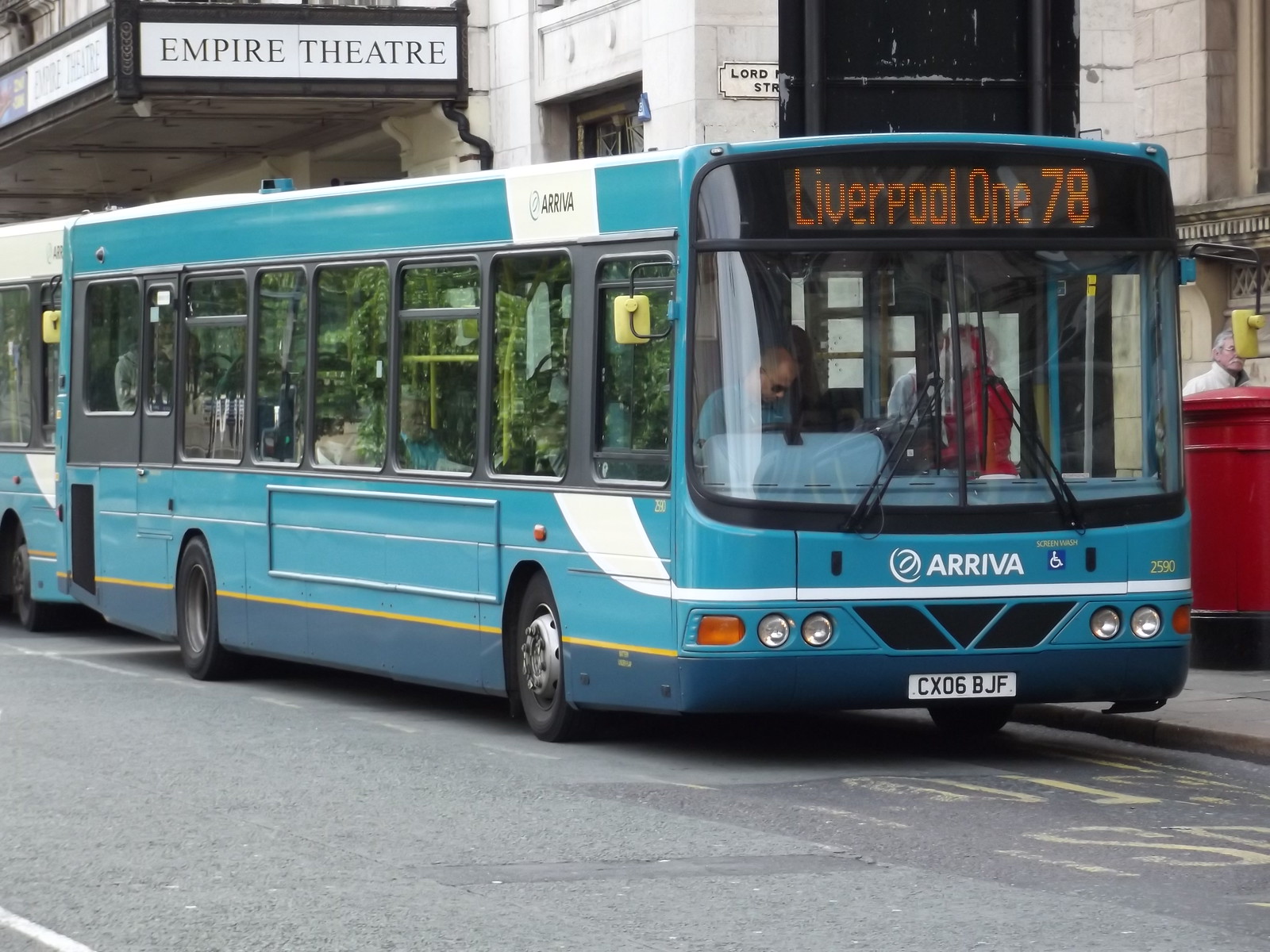The image depicts a city scene in England, featuring two blue city buses parked side by side along the sidewalk against a building. The bus in the foreground, a light blue, one-story bus with about eight black-framed windows, prominently displays "Liverpool 178" in orange text on its digital sign at the top front. The bus also bears the company name "Arriva" in white text at the bottom front, and its license plate reads CX06BJF. Through the front window of this bus, a lady in red is visible on the other side. The bus driver, wearing sunglasses, is seen looking down, and the bus is stationary.

The scene includes additional elements: above the buses, the facade of a building displays a sign reading "Empire Theatre." On the right side of the image, there is a red feature of the building next to the sidewalk, with a man in a white shirt standing nearby. The overall weather appears clear with dry pavement, indicating it is not raining.